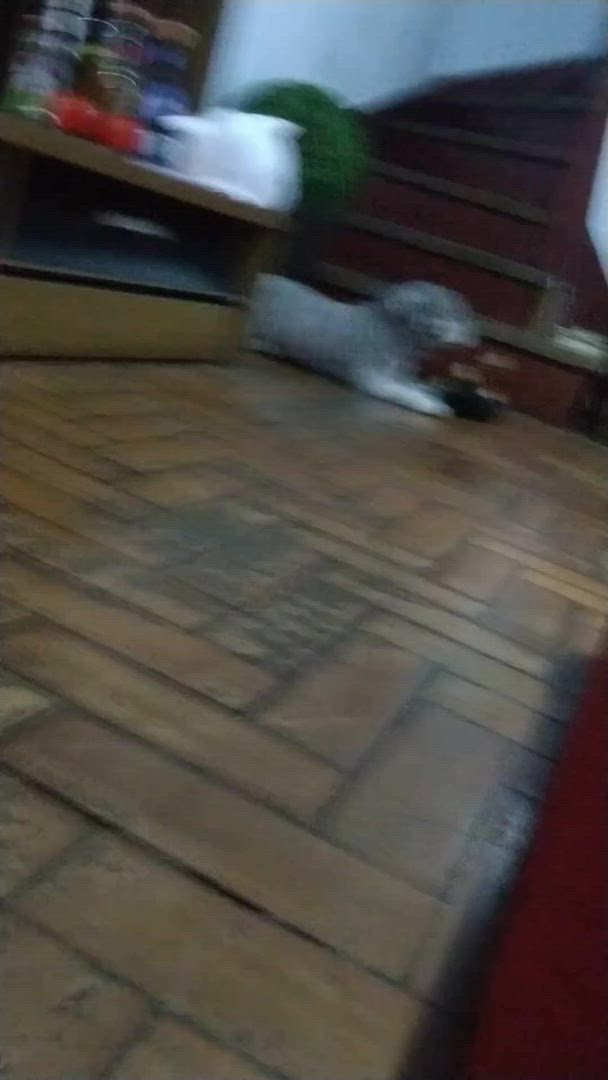The image is a slightly blurry, rectangular photograph of a grey-colored dog lying on its stomach. The photo captures an angled perspective, with the top of the setting pointing toward the top right corner and the bottom toward the bottom left corner. The room features a zigzag-patterned floor made of rectangular brown bricks, separated by black grout lines. A red-painted wall is visible in the bottom right corner. In the top left corner, there is a light brown cabinet featuring a black drawer at the bottom and a large shelf with a plastic bag and three bottles on top. Positioned behind the cabinet, the dog reclines in front of a set of red and black steps that lead upwards, contributing to the complex, textured environment of the image.